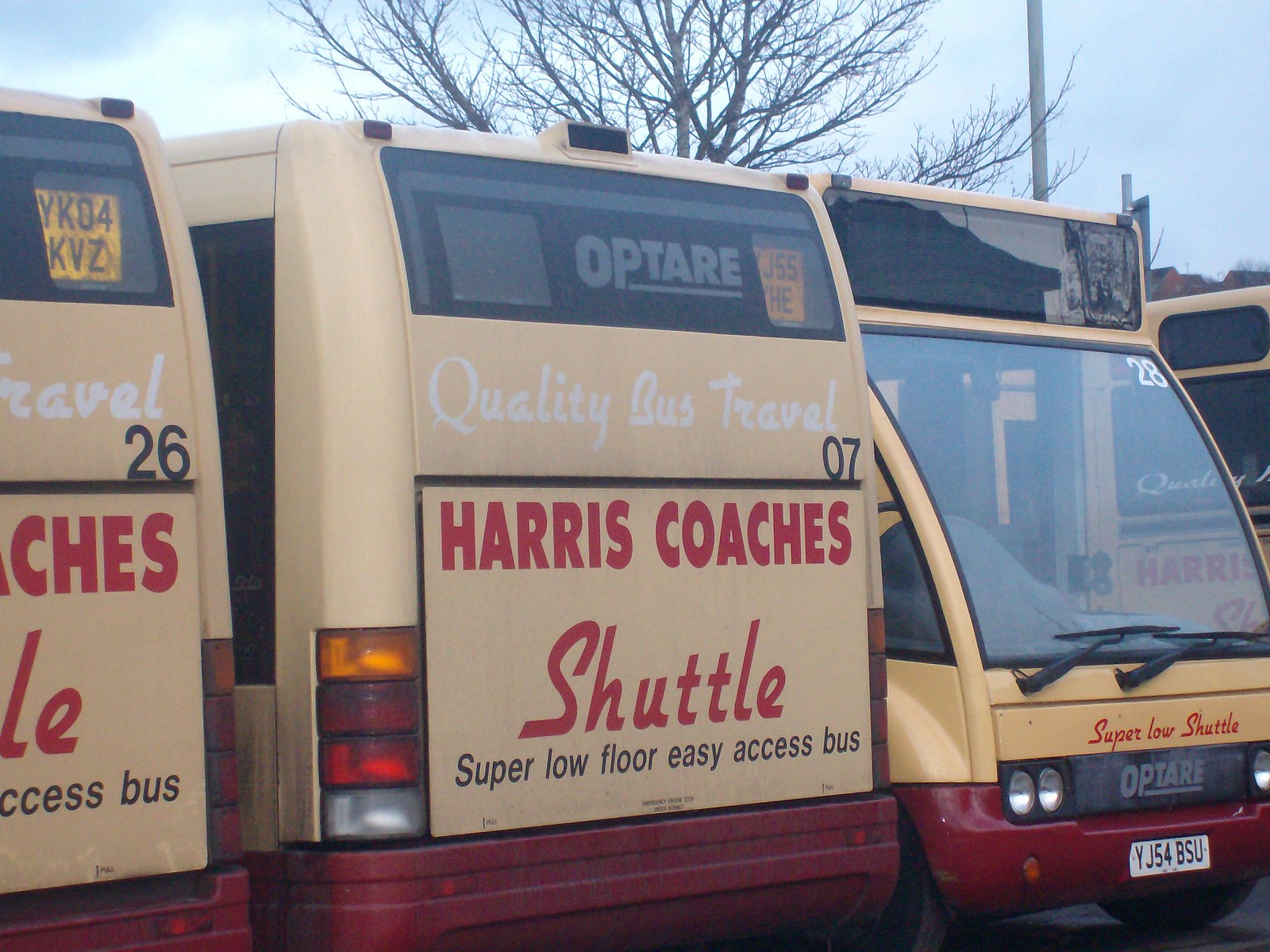In this outdoor photograph, four red and yellow Harris Coaches shuttle buses are lined up in a parking lot under an overcast sky, accented with patches of blue and white clouds. The scene also features a large bare tree with no leaves and a thin pole to the right. The buses prominently display "Quality Bus Travel," "Super Low Floor Easy Access Bus," and the "Harris Coaches" logo. The first bus, numbered 26, and the second bus, numbered 07, are fully visible, while the third bus, numbered 28, and the fourth bus are partially obscured. The third bus has a license plate reading YJ54 BSU and displays "Optair" on it. More buses are seen parked in the distance, adding depth to the image.